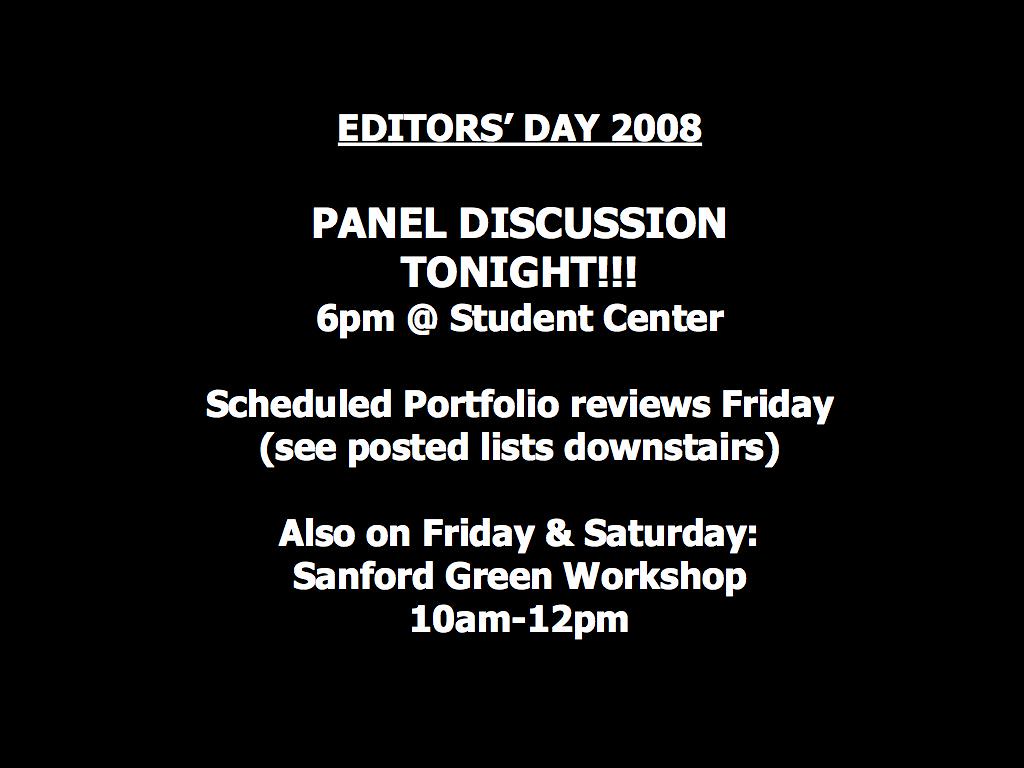The image features centered white text on a black background in what appears to be the Tahoma font. At the top, in large, underlined, all-caps text, it reads "EDITORS DAY 2008." Just below, also in all caps, it announces, "PANEL DISCUSSION TONIGHT!!!" The event's time and location follow in mixed case: "6 p.m. at Student Center." Beneath this, in regular capitalization, there's information about scheduled portfolio reviews on Friday, instructing viewers to "see posted lists downstairs." Finally, it mentions a workshop: "Also on Friday and Saturday: Sanford Greene Workshop, 10 a.m. to 12 p.m."